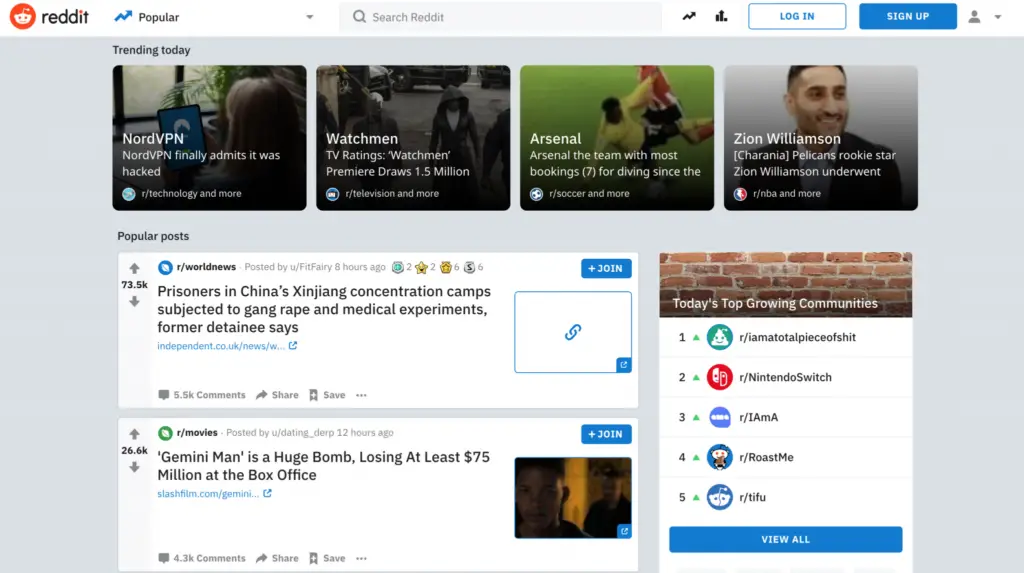The image depicts the homepage of the Reddit website. Prominently displayed on the top-left of the page is Reddit’s logo, featuring the iconic alien mascot known as "Snoo." To the right of this logo is a menu for trending topics. 

Highlighted under the "Trending Today" section are four key stories:
1. Norton VPN admits to a hacking incident, detailing the breach.
2. The TV series "Watchmen," which premiered with 1.5 million viewers.
3. Arsenal F.C., infamous for receiving the highest number of bookings for diving in soccer.
4. Zion Williamson, the rookie star for the New Orleans Pelicans, who has undergone surgery due to a recurring injury since leaving Duke University.

Additionally, the website features a search bar for browsing topics and a login/sign-up option for those with a Reddit account. 

Below the trending topics, there are sections for popular posts and growing communities. One popular post from World News discusses the harrowing conditions in China's Xinjiang concentration camps, describing instances of gang rape and medical experiments as reported by a former detainee. Another post reviews the film "Gemini Man," noting its significant financial loss of at least $75 million at the box office.

The image also includes a section for exploring other growing subreddit communities, with a list of the top five trending communities and an option to view more. 

Overall, the picture outlines the main features and current hot topics on Reddit's homepage, emphasizing the site's extensive content ranging from global news to entertainment and sports.